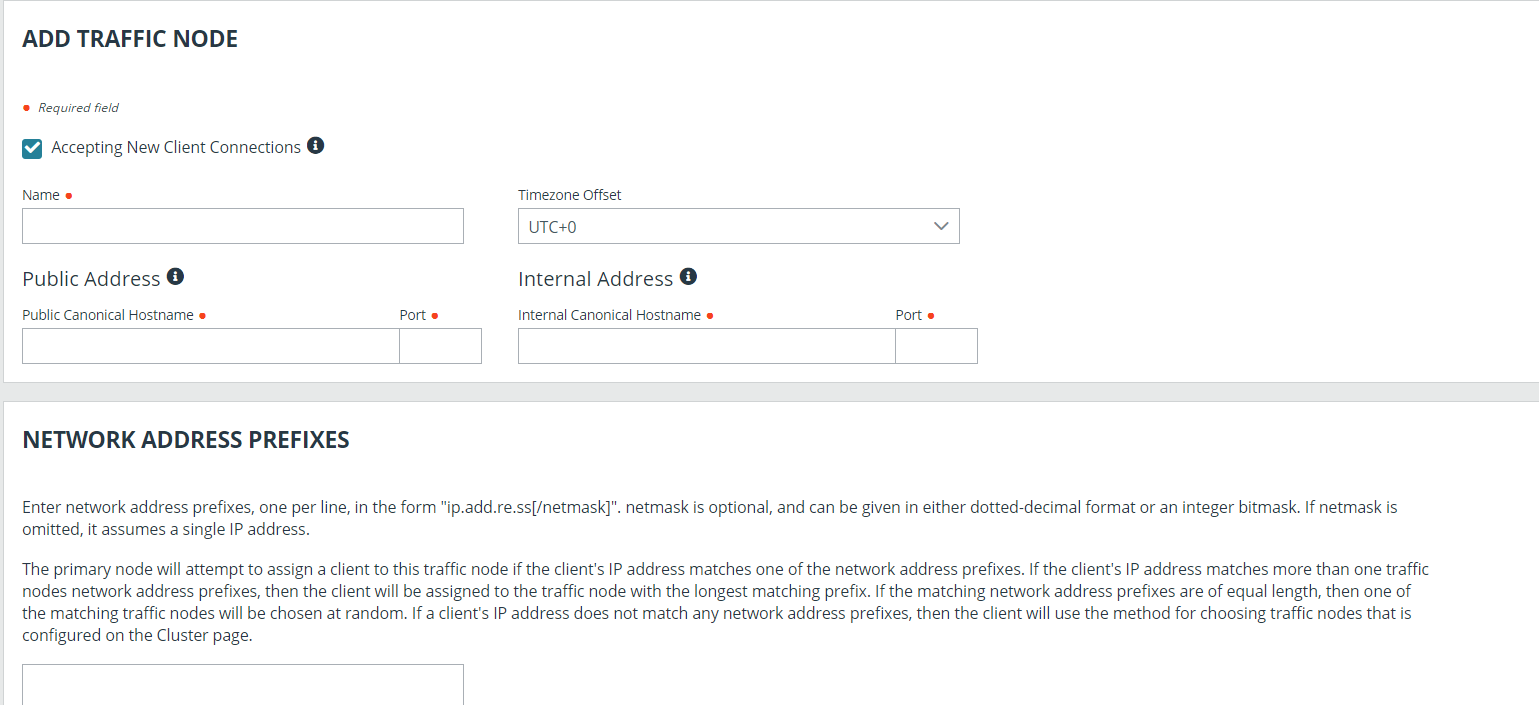The screenshot displays a form titled "Add Traffic Node" located in the upper left-hand corner of the image. A red asterisk beside the title indicates that certain fields are required. Below this, a checkbox labeled "Accepting New Client Connections" is visible.

The form features multiple sections. The first section, marked by the label "Name," contains a blank text box intended for the user to input a name. Adjacent to this, there's a "Time Zone Offset" field accompanied by a dropdown menu set to "UTC+0."

In the lower portion of the form, the "Public Address" section includes a text box for entering the Public Connection Host Name and a separate box for the port number. To the right of this, the "Internal Address" section mirrors the format with identical text boxes for internal addressing details.

The next section, titled "Network Address Prefixes," consists of two lines of text explaining relevant information about network address configurations. Although the text is small and somewhat difficult to read, it gives users necessary details for filling out the form correctly.

Finally, at the very bottom left-hand corner of the form, there is another blank text box, serving an unspecified purpose, awaiting user input.